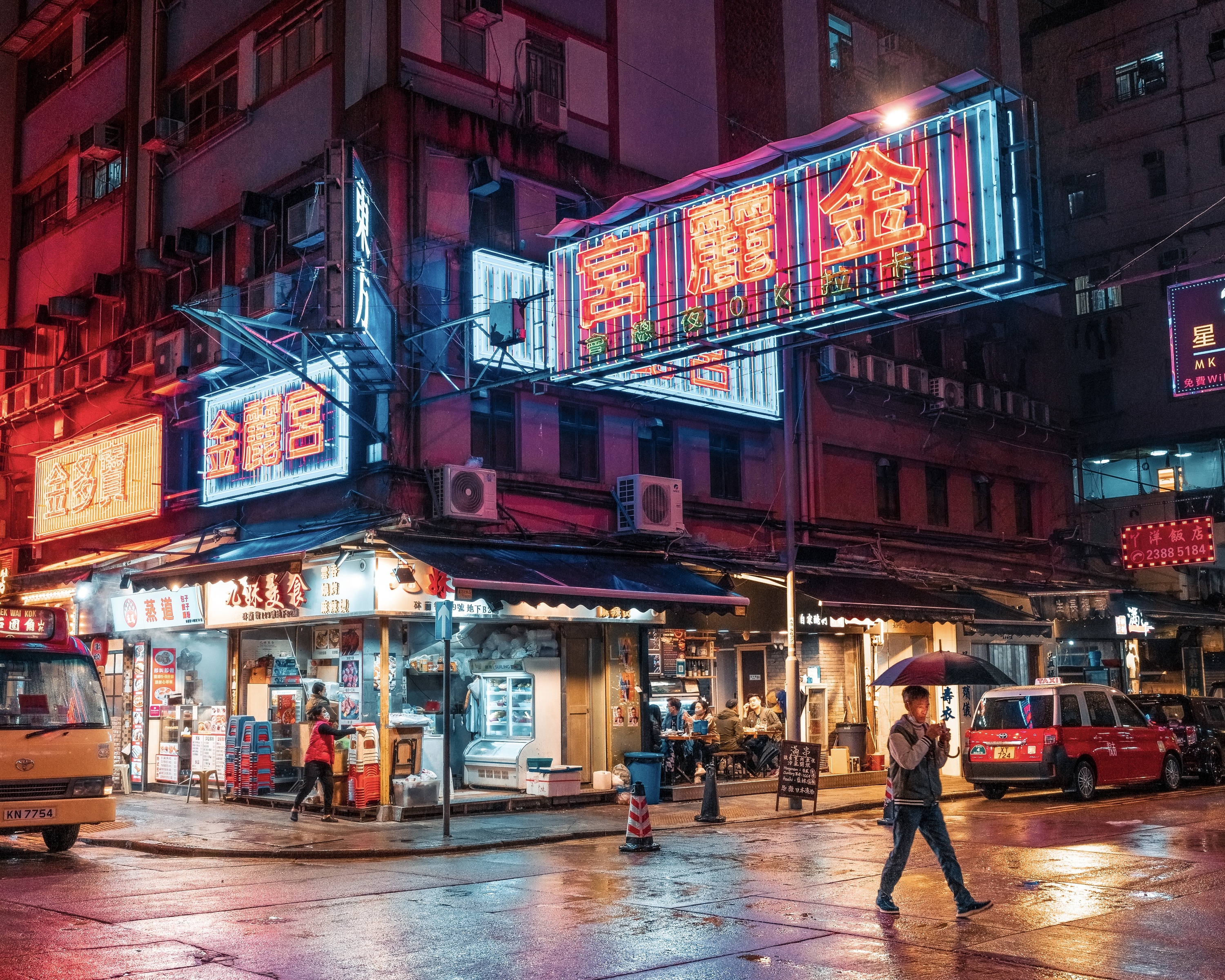The scene is a vibrant nighttime street in what appears to be Tokyo or a major Japanese city, bathed in a futuristic, neon glow. Brightly lit signs with Japanese characters illuminate the tall apartment buildings and bustling city streets. Reflections dance on the wet sidewalk, adding to the surreal atmosphere. The rain is evident from the man walking towards the camera while engrossed in his phone, holding an umbrella. On the left side, a Toyota, which could be a taxi or bus, approaches, while on the right, a small red and white car is parked. In front of various lit-up businesses, people are seen dining in small restaurants or cafeterias, and a child in a red vest stands at the corner. The entire scene, captured with professional precision, evokes a sense of urban life in a sprawling Asian metropolis.